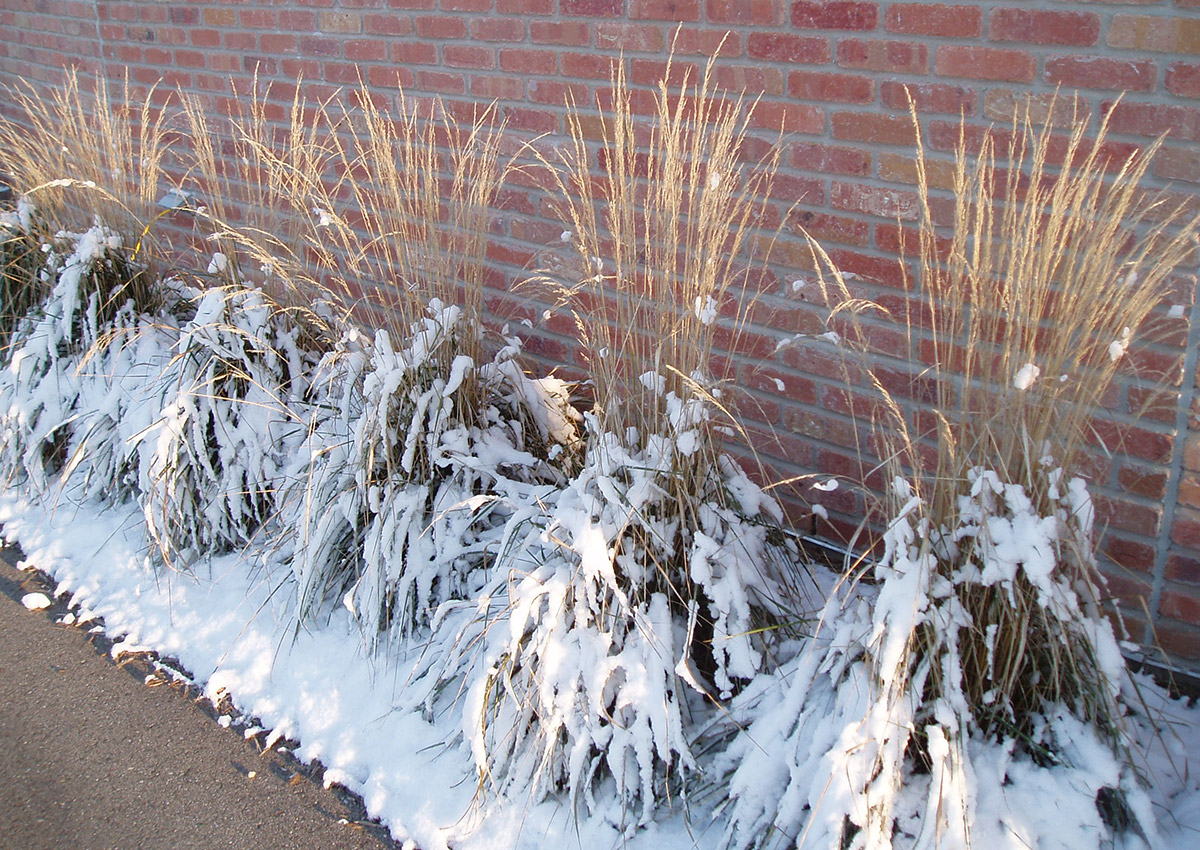The photograph captures a picturesque outdoor scene featuring tall decorative grasses planted along a red brick wall with grey mortar. The grasses, which have brown tops, are partially covered with snow at their bases, and snow has banked up around them throughout the flower bed. Sunlight glints off the tops of the grasses, casting the lower portions in shadow. In the bottom left-hand corner, a section of dark, grey paved surface—possibly a sidewalk or driveway—can be seen. The overall image is well-lit, showcasing the contrast between the snowy ground and sunlit plants against the decorative brick backdrop.